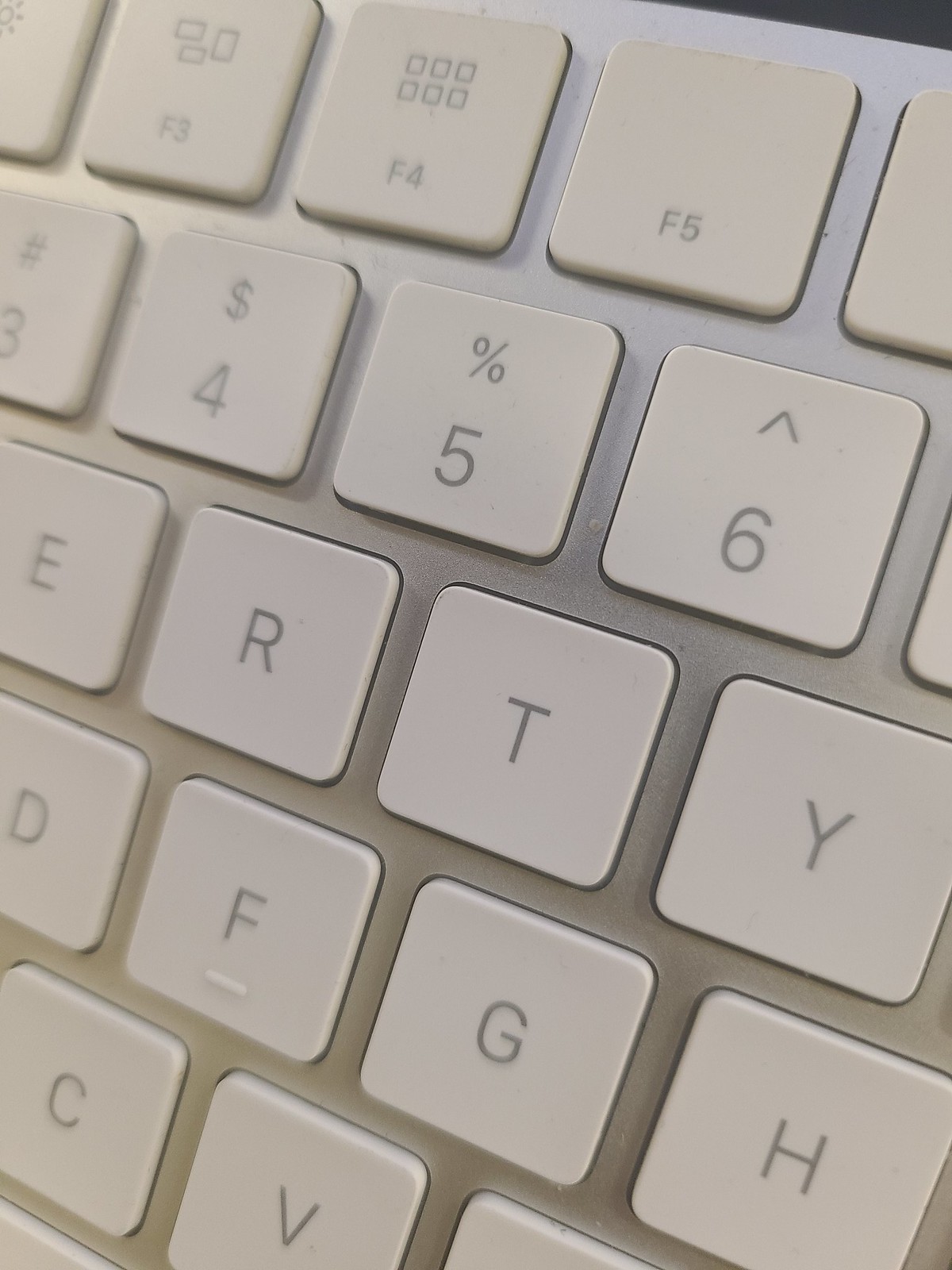The image showcases an extremely close-up view of a segment of a laptop keyboard, highlighting its distinct flat, light gray keys against a silver background. At the very top, we notice the function keys: F3 with three small squares, F4 with two rows of three squares each, and F5 devoid of any symbols. Just below, the number keys are visible: the 3 key featuring a hashtag, the 4 key with a dollar symbol, the 5 key displaying a percent sign, and the 6 key marked by an upward-pointing caret. Further down, sequential rows reveal the letters E, R, T, Y; D, F, G, H; followed by C, V, and a barely visible B key. The keys, with darker gray characters, appear slightly dirty. The framing is so zoomed in, it captures only a fraction of the keyboard, with just a small sliver of a black background visible at the top right corner.